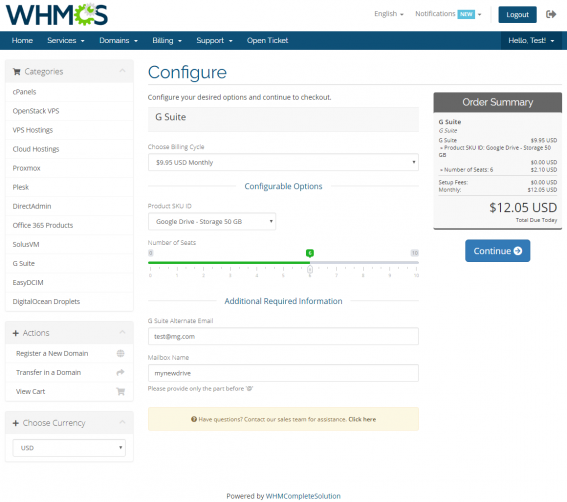The screenshot depicts a detailed interface of a web hosting management website. The page features a clean, white background with the header prominently displaying "WHM" in capital letters, followed by a gear icon that resembles the letter "C", and then an "s" to form the "WHMCS" logo. 

To the right of the logo, the interface offers a language selection option currently set to "English" with a downward arrow for additional choices. This is followed by a notifications section indicated by a blue square with the word "new" in white text within a dropdown menu. Adjacent to this, there's a "Log Out" button with a navy blue background and white text.

Below the header, there is a blue horizontal banner that houses the main navigation menu. This menu includes options like "Home", "Services" (with a dropdown), "Domains" (with a dropdown), "Billing" (with a dropdown), and "Support" (with a dropdown). Further along the menu, there's an "Open Ticket" option and a greeting, "Hello, Test!", accompanied by a dropdown marked by an exclamation point.

The main section features a white background and provides instructions: "Configure your desired options and continue to checkout." Below this, it lists options related to "G Suite". Users can select the billing cycle, configure options, and input the number of seats along with any additional required information.

On the right side of the main section, there's an "Order Summary" box detailing the summary of the G Suite order. It shows an item, "G Suite," priced at $9.95 USD per seat. The summary indicates an order of six seats with setup fees and calculates a total due today of $120.05. 

A prominent "Continue" button in blue with white text is located at the bottom for proceeding with the order. Finally, the left sidebar lists various categories: Panels, OpenStack VPS Hostings, Cloud Hostings, Pro Max, Plesk, Direct Admin, Office 365, Products, SolusVM, G Suite, Easy DC, IAM, and Digital Ocean Droplets, allowing users to navigate other services and products offered by the website.